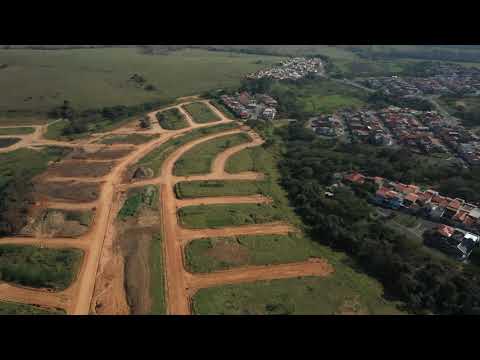This aerial photograph captures a sprawling landscape with a blend of natural and developed areas, framed by two horizontal black lines at the top and bottom, giving it a screenshot-like appearance. The central focus of the image reveals a field marked by several brown dirt tracks forming parallel and perpendicular lines, indicating a housing subdivision under construction. The unpaved roadbeds of this developing area create a network of main roads and branching cul-de-sacs, interspersed with verdant patches of green grass yet to be built upon. Off to the right, a similar but fully developed subdivision mirrors this pattern, with houses neatly lining the cul-de-sacs and green spaces populated with trees. In the foreground, vibrant green fields dominate the scenery, while smaller green plants and larger trees dot the landscape. Beyond the immediate foreground, clusters of neighborhoods with some red-roofed buildings stretch out, although the haziness of the image renders the finer details and street layouts indistinguishable. The sun is visibly shining, enhancing the daytime atmosphere, but the overall image remains slightly blurry. Notably, there are no people or automobiles visible in this serene and expansive vista.